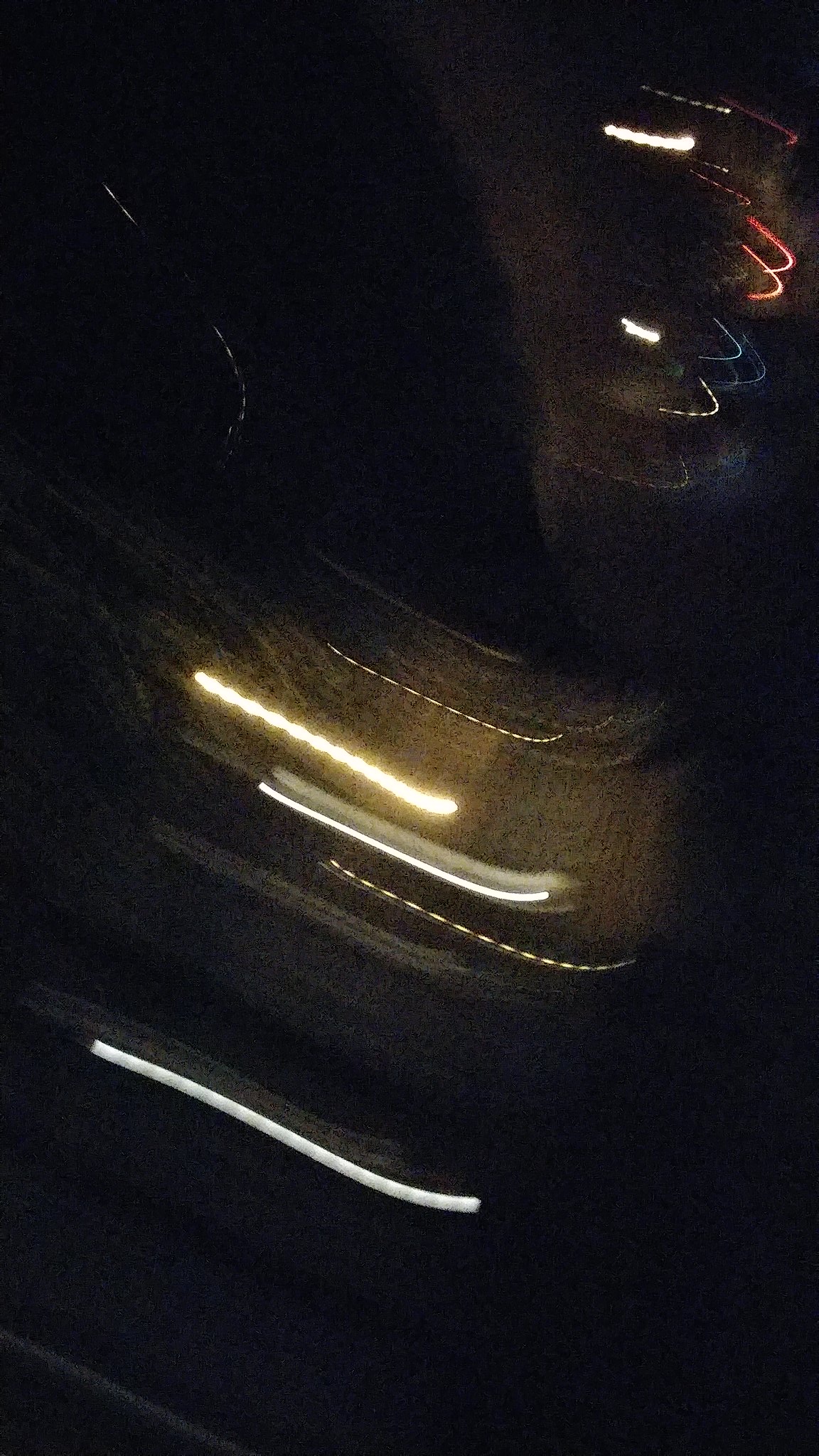Caption: 

A chaotic and intriguing photo captures the interior of a car illuminated by the flash, creating a complex interplay of lights and reflections. The flash has produced multiple linear reflections—three of which are bright, white lights—adding to the confusion and mirroring effect on the car's surfaces. In addition, the image showcases around five more lights that range in color from red to blue, adding a splash of vibrant hues against the dark background. The black foreground and background seem to blend into each other, vaguely revealing seating arrangements and wires, further obfuscating the scene but adding to its mysterious allure.